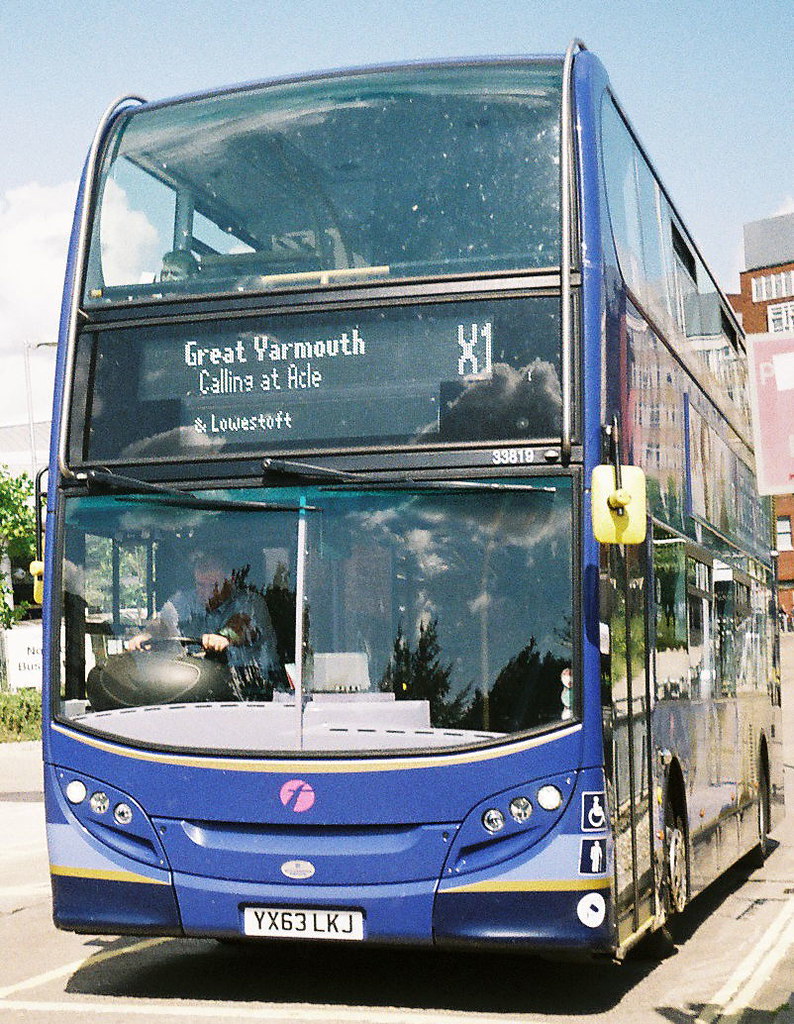The photograph captures a large blue double-decker bus taking up the majority of the image, set against a backdrop of a sunny sky with a few clouds. To the sides, you can see some buildings and a bit of foliage. The bus, distinguishably marked with the license plate YX63LKJ, features yellow rearview mirrors and prominently displays its destination on a front visual sign: "Great Yarmouth, calling at ACLE," alongside a large "X1" and a smaller text reading "Lowestoft."

The bus number, 33819, is visible at the top right of the windshield. Inside, on the left-hand side, the male driver wearing a blue collared shirt is holding the steering wheel, looking ahead. A single passenger’s head is faintly visible at the top left of the bus’s interior. The sun casts a bright light, illuminating the ground prominently.